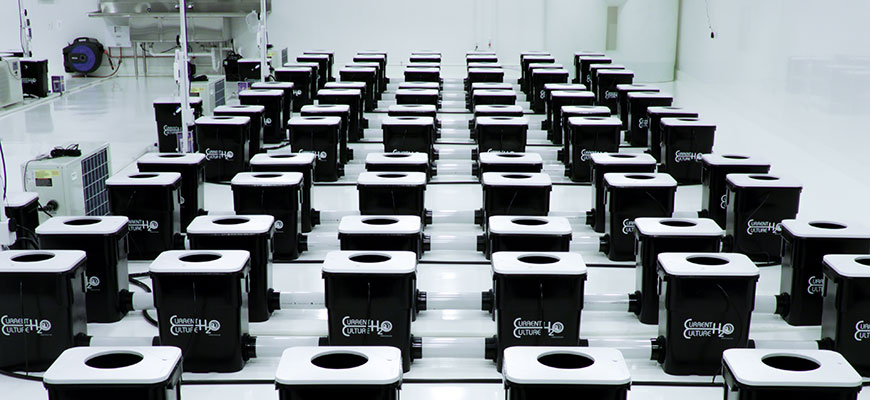This indoor photograph, likely taken in a sterile lab environment, features white walls and a pristine white floor. The central focus is on six rows of neatly arranged black canisters with white lids, each featuring small circular holes. In total, there appear to be around 20 canisters per row, though some sources suggest variations in count per row. Small, hard-to-read white writing on these canisters possibly indicates they are used for water purification or another industrial process. Towards the back, there's a larger industrial machine that is black with blue elements, accompanied by at least two large white air conditioning units. The left side of the image also reveals additional equipment, possibly metal shelving holding a silver machine, adding to the complex and technical setup of the space. The overall arrangement suggests a highly organized and purposeful layout, characteristic of a specialized lab or workspace.